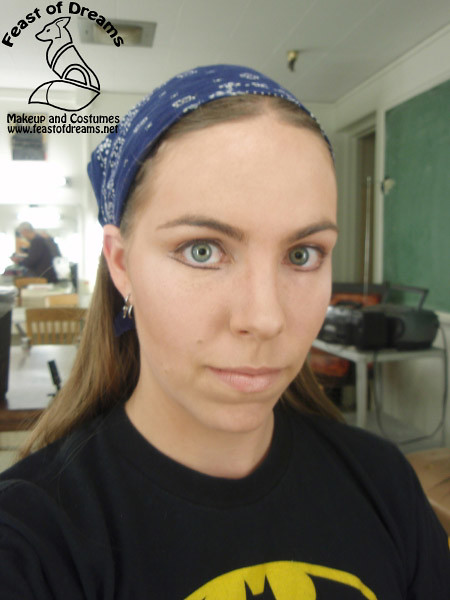The image is a detailed, color portrait photograph taken as a cell phone selfie in portrait orientation. It features a young woman, approximately 22 years old, with long brown hair held back by a blue bandana, making her green eyes and slight pink-lipsticked smile stand out. She is wearing a black t-shirt emblazoned with the yellow Batman logo. The woman is centrally positioned, looking directly at the camera with a hint of black eye makeup and earrings, conveying a mix of confidence and subtle discomfort. 

In the background, an interior room that resembles a makeup studio is visible, distinguished by white walls, a green chalkboard, and a boombox among other equipment. The top left corner of the image prominently displays the logo for "Feast of Dreams," accompanied by an illustration of a fox and text advertising "Makeup and costumes, www.feastofdreams.net." Other people and furniture are present in the background, but they are out of focus, ensuring the viewer's attention remains on the woman. The style is realistic and typical of a contemporary cell phone selfie.